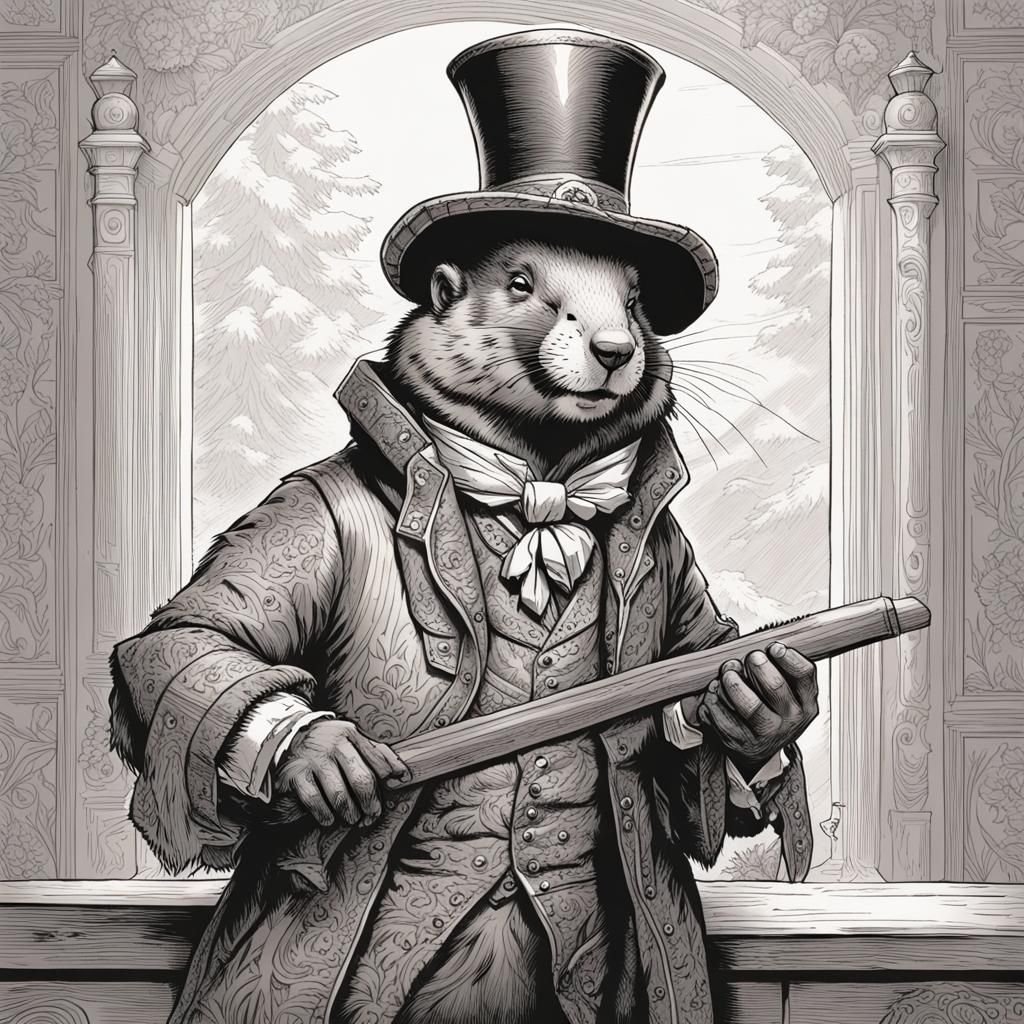The image is a highly detailed black and white illustration of an anthropomorphic groundhog, resembling an aristocratic figure. The groundhog is centrally positioned, looking directly at the viewer. It is intricately dressed in a vintage suit that includes a long embroidered coat, a matching vest with fine detailing, a collared shirt, and a white scarf tied in a bow. Completing its dapper look, the groundhog wears a shiny black top hat. It holds a stick-like object in its human-like fingers.

The background features an arched window that opens to an outdoor scene, showcasing a pale, possibly cloudy sky with visible power lines, and two conifer trees. This window is flanked by gray pillars. The walls surrounding the window are detailed with an intricate pattern and wainscoting, adding to the illustration's vintage charm. There’s also a wooden ledge at the bottom of the image against which the groundhog appears to be leaning.